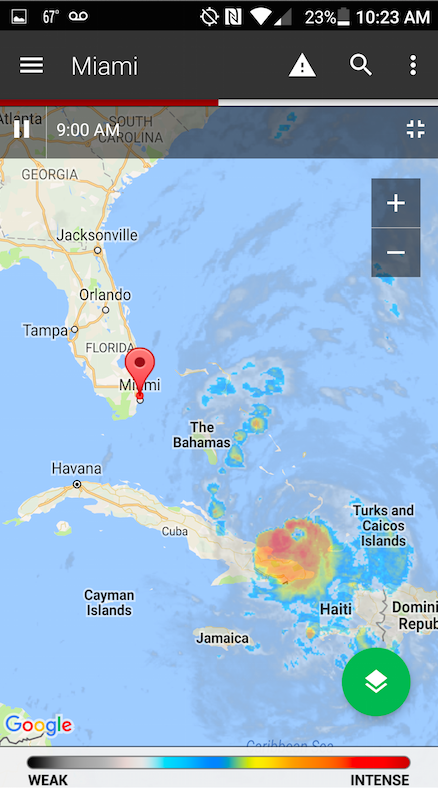In this vertically oriented rectangular image, which appears to be a snapshot taken from a phone, the top of the image features a black border running horizontally across the screen. This border contains a series of icons, including a mountainscape, a temperature reading indicating 67 degrees, various unrecognized symbols, a full-strength Wi-Fi signal, a cell signal showing two bars, a battery indicator at 23% usage, and the current time displayed as 10:23 AM.

Below this black border, another gray horizontal strip is present. On the left side of this strip is a hamburger menu symbol, followed by the label "Miami" in the center. To the right of "Miami" is a magnifying glass icon for the search, and three vertically aligned dots on the far right.

The main section of the image displays a map that includes the entire state of Florida, portions of Georgia and South Carolina, and several nearby islands. A pin marks the location of Miami. Also depicted are the Bahamas, Cuba, Haiti, the Dominican Republic, Jamaica, the Cayman Islands, and the Turks and Caicos Islands. Dominating the latter part of the image is a weather map that appears to show the development of a tropical storm moving over Cuba.